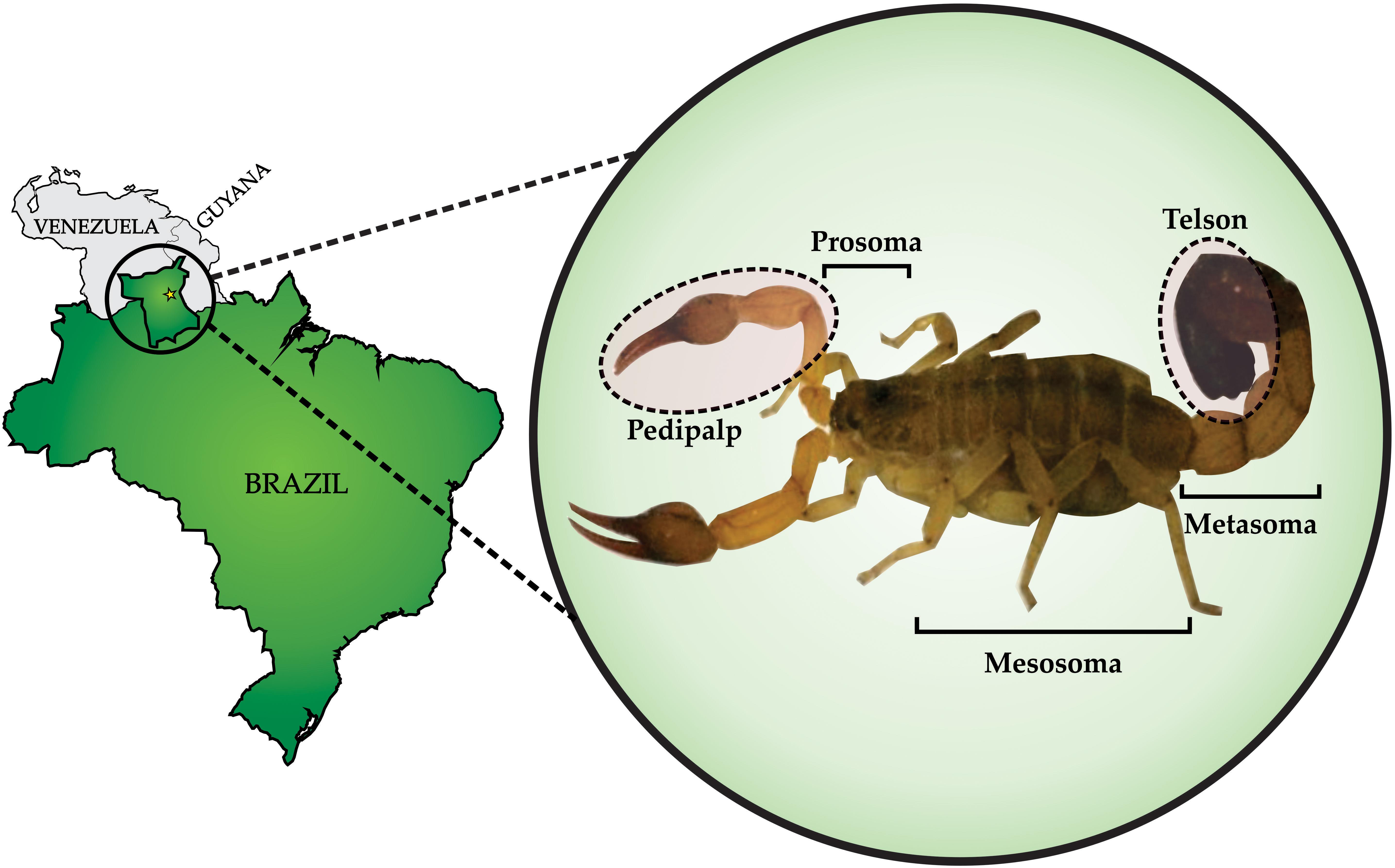This infographic features a detailed illustration of a scorpion with labeled anatomical parts. The scorpion is shown in a light green circle on the right side of the image, with its body parts meticulously outlined and identified. The right claw is labeled as a "pedipalp," the upper body is labeled "prosoma," the midsection is detailed as "mesosoma," the tail is referred to as "metasoma," and the stinger at the end of the tail is marked as "telson."

On the left side of the image, there is a green color-coded map highlighting Brazil, with neighboring Venezuela and Guyana also visible. A specific region within Brazil is circled, and a star marks the precise location where this scorpion species can be found, indicating its habitat. The corresponding region on the map is connected by dotted lines to the circle containing the scorpion specimen, illustrating the geographic context of the species.